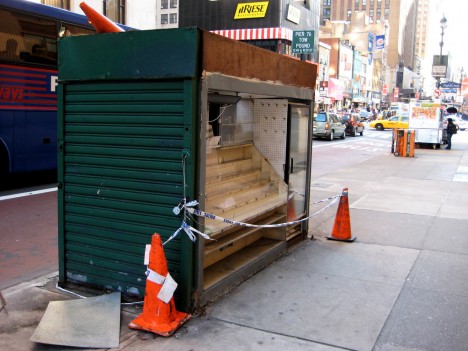A bustling daytime scene captures a typical New York City sidewalk, dominated by a prominent, tall rectangular newsstand on the left side, partially obscured by a padlocked green metal gate and flanked by orange safety cones with white and blue caution tape. The newsstand appears abandoned, with open shelves and a small glass-door refrigerator at the front. The sidewalk, paved with large gray stones, leads into a busy street populated with a yellow taxi and a bus with blue and red horizontal stripes. There's a hot dog vendor in the distance, reinforcing the city's vibrant street life. Overhead, several tall buildings frame the scene, hinting at a location possibly around Times Square or Madison Square Garden, as suggested by nearby blue street signs and other city landmarks. The sidewalk features a mix of pedestrians and traffic, including a city bus and bustling cars, underscoring the lively, chaotic energy of New York City. In the background, a yellow sign on a building spells out "D-R-I-E-S-E," adding to the detailed urban tapestry of the scene.